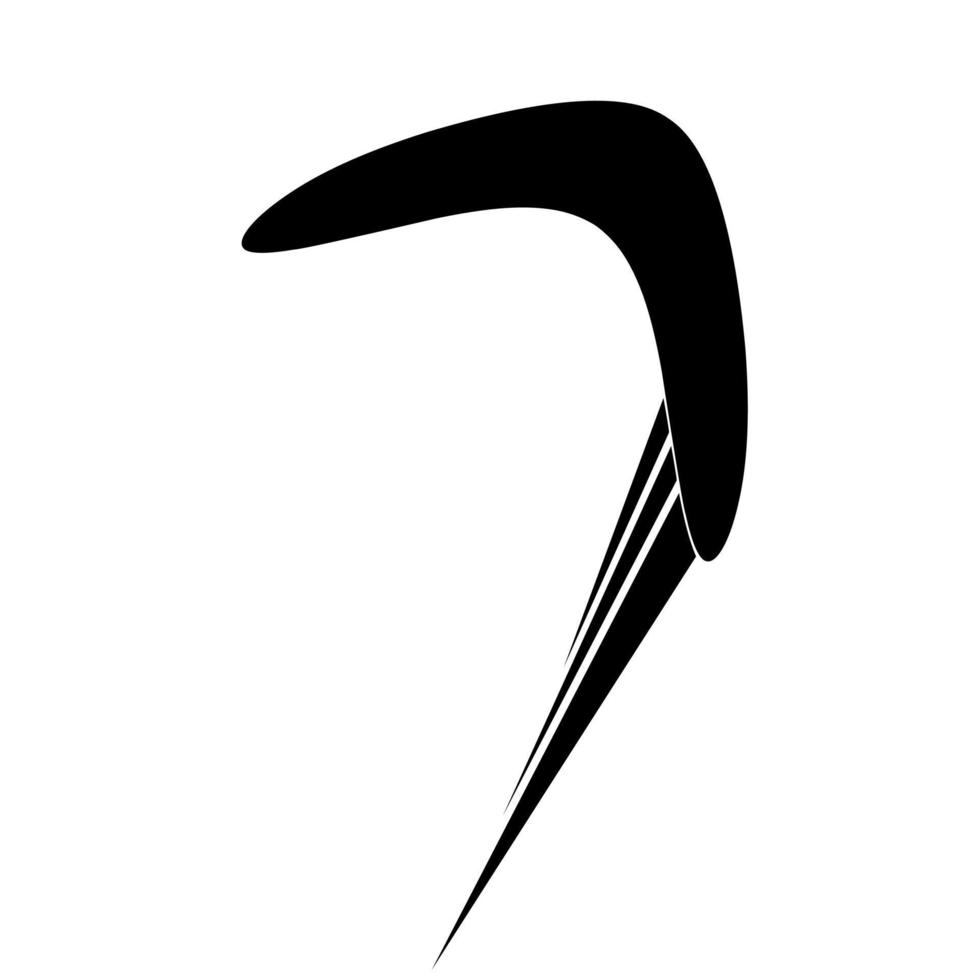The image features a simple black and white design, with a stark white background serving as the canvas. The centerpiece is a black, right-angled boomerang clip art graphic that faces upward at an angle toward the upper right corner of the image. The boomerang appears as though it has been thrown, with three long, tapering black streaks trailing off its right side, suggesting its rapid movement through the air. These streaks, all uniformly black like the boomerang, indicate motion and speed: the longest streak is at the bottom, the middle one slightly shorter, and the top one the smallest. Small white spaces separate each streak, emphasizing the dynamic path of the boomerang against the minimalist white background.